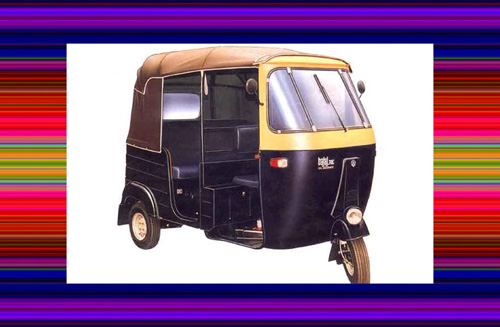This full-color, computer-generated digital image is rectangular with horizontal long edges and vertical short edges. The background features a vibrant pattern of horizontal stripes in various colors, including blues, purples, reds, oranges, yellows, and greens, creating a rainbow-like gradient frame around the central subject. The focal point of the image is a digital representation of a tuk-tuk— a three-wheel vehicle commonly used as a taxi in Taiwan or Thailand. This motorized tricycle has a single front wheel equipped with a headlight, and two smaller wheels at the rear. It features a canvas top in a beige hue, and the body has a blue base with yellow trim around the windows. The windshield is opaque but includes visible windshield wipers and side mirrors on both sides. The vehicle is depicted on a flat white background, accentuating its details and colors while the entire scene is devoid of any human presence.